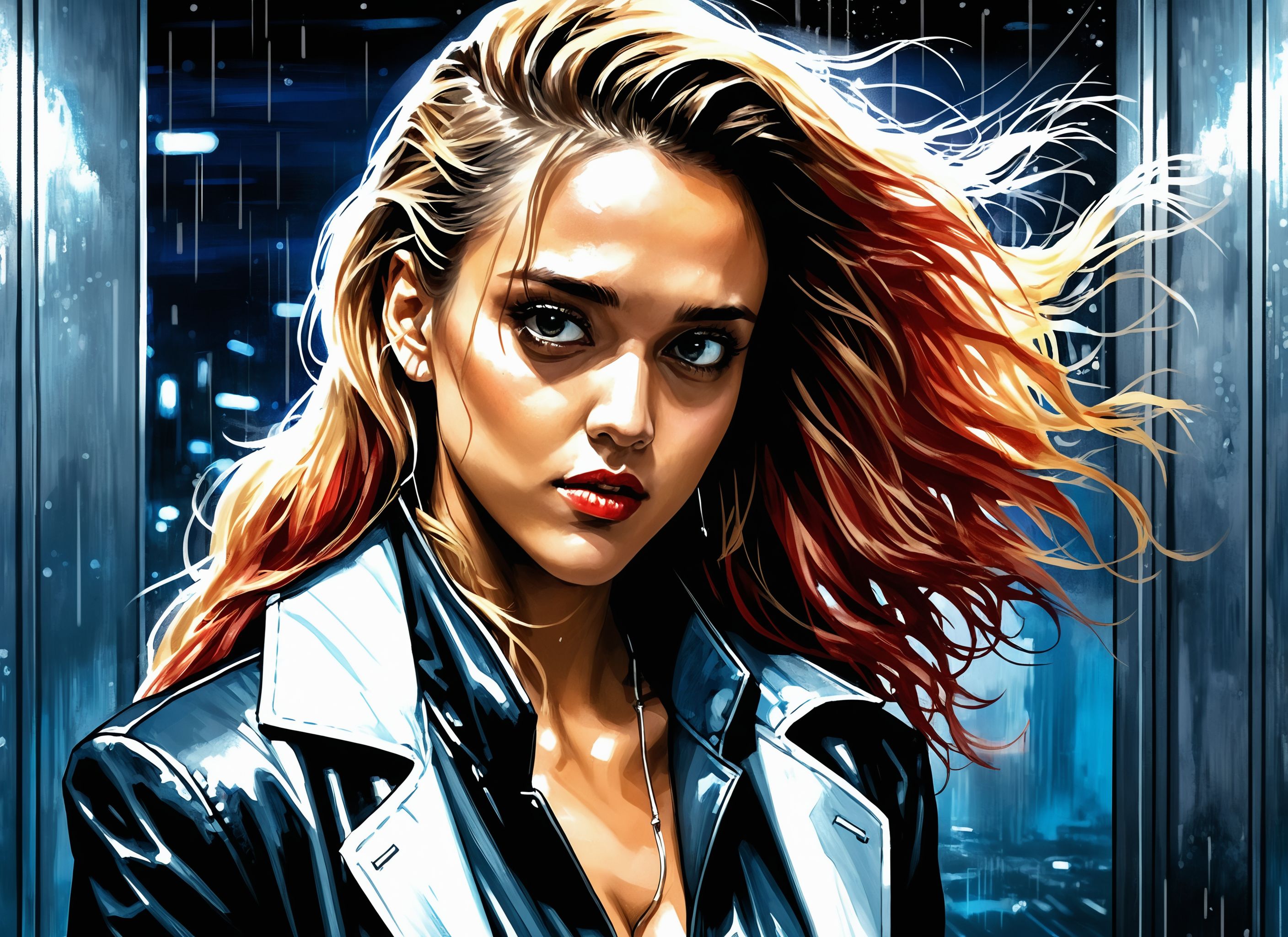This digital art piece depicts an animated female character, likely in her late teens or early twenties, exuding a striking visual presence. She is characterized by her long hair, which transitions from a base of blondish-brown to reddish tips, blowing gently to the right. Her hair is parted on the side, and she sports dark red lipstick on her slightly open, full lips. She has large, expressive gray eyes with shadows framing them, and her gaze is directed straight at the viewer.

She is adorned in a black leather jacket, complete with a detailed, folded collar that appears gray. Underneath, she wears another jacket of a similar material. A distinct silver chain necklace hangs around her neck, subtly extending into her outfit. The image captures her from just below the shoulders upwards.

The background hints at a setting beyond the immediate focus, featuring blurry vertical gray streaks suggesting rain against a window. There are also silhouettes of city buildings visible through the window's sleek, shiny frame, and dark doors with glass panels, adding depth and urban ambiance to the scene. The image's landscape layout frames the character centrally, enhancing her presence in a visually compelling manner.